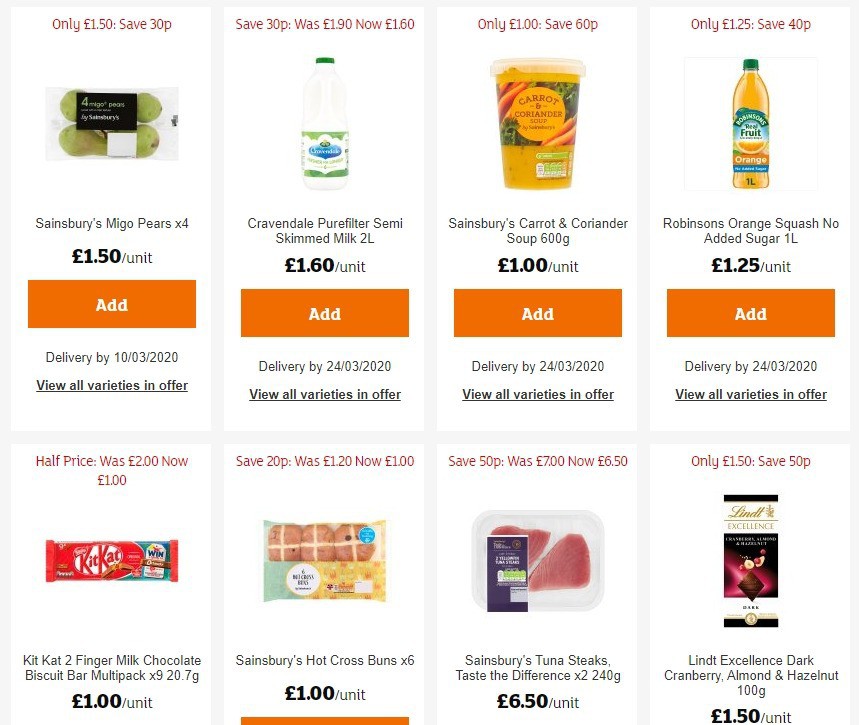**Detailed Caption:**

This is a detailed screenshot of a grocery shopping app interface. The display features two rows of product listings, each containing four items. 

In the top row, the first item is "Sainsbury's Mango Pears," priced at £1.50 per unit. The second item listed is "Cravendale Pure Filter Semi-Skim Milk," available in a 2-liter bottle for £1.60 per unit. The third item is "Sainsbury's Carrot and Coriander Soup," weighing 600 grams and priced at £1.00 per unit. The fourth and final item in this row is "Robinson's Orange Squash," boasting a no-added-sugar formula in a 1-liter bottle for £1.25 per unit. Each product box features an orange "Add" button with white text.

The lower row showcases four more items. The first is a "KitKat 2 Finger Milk Chocolate Biscuit Bar Multi-Pack," priced at £1.00 per unit. The next item is a pack of "Sainsbury's Hot Cross Buns," containing six pieces, also priced at £1.00 per unit. Following that is "Sainsbury's Tuna Steaks," with a total weight of 240 grams, priced at £6.50 per unit. The final item in this row is "Lindt Excellence Dark Cranberry Almond and Hazelnut," a 100-gram bar available for £1.50 per unit. 

Each of these items is accompanied by an "Add" button in orange, featuring white lettering for easy product addition to the cart.